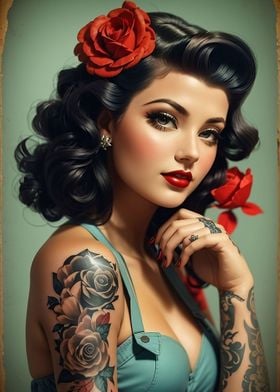In this richly colored, vintage-inspired image, a young brunette woman, approximately 18 years old, gazes towards the camera with a captivating, seductive expression. Her shoulder-length, curly, dark brunette hair is styled in intricate, pinned-up curls typically seen in pin-up models, adorned with red roses—one positioned above her right ear and another faintly visible on the left. Her light blue eyes are set against the backdrop of her flawless skin, accentuated by dark eyebrows, bold ruby red lipstick, heavy eye makeup, and a touch of blush.

She dons a low-cut, smoky blue halter top that reveals an elaborate rose tattoo on her right shoulder, featuring both dark and light hues. Her left hand, decorated with tattoos on the fingers and forearm, is elegantly curled up towards her cheek, showcasing her extensive and intricate body art, which includes roses on her upper bicep and shoulder.

The background is a soft, light green, contrasting with her striking features and the grayscale hues of her dress, enhancing the overall vintage aesthetic of the image. Her look is completed with small stud earrings, adding a subtle touch of elegance to her bold and classic pin-up style.